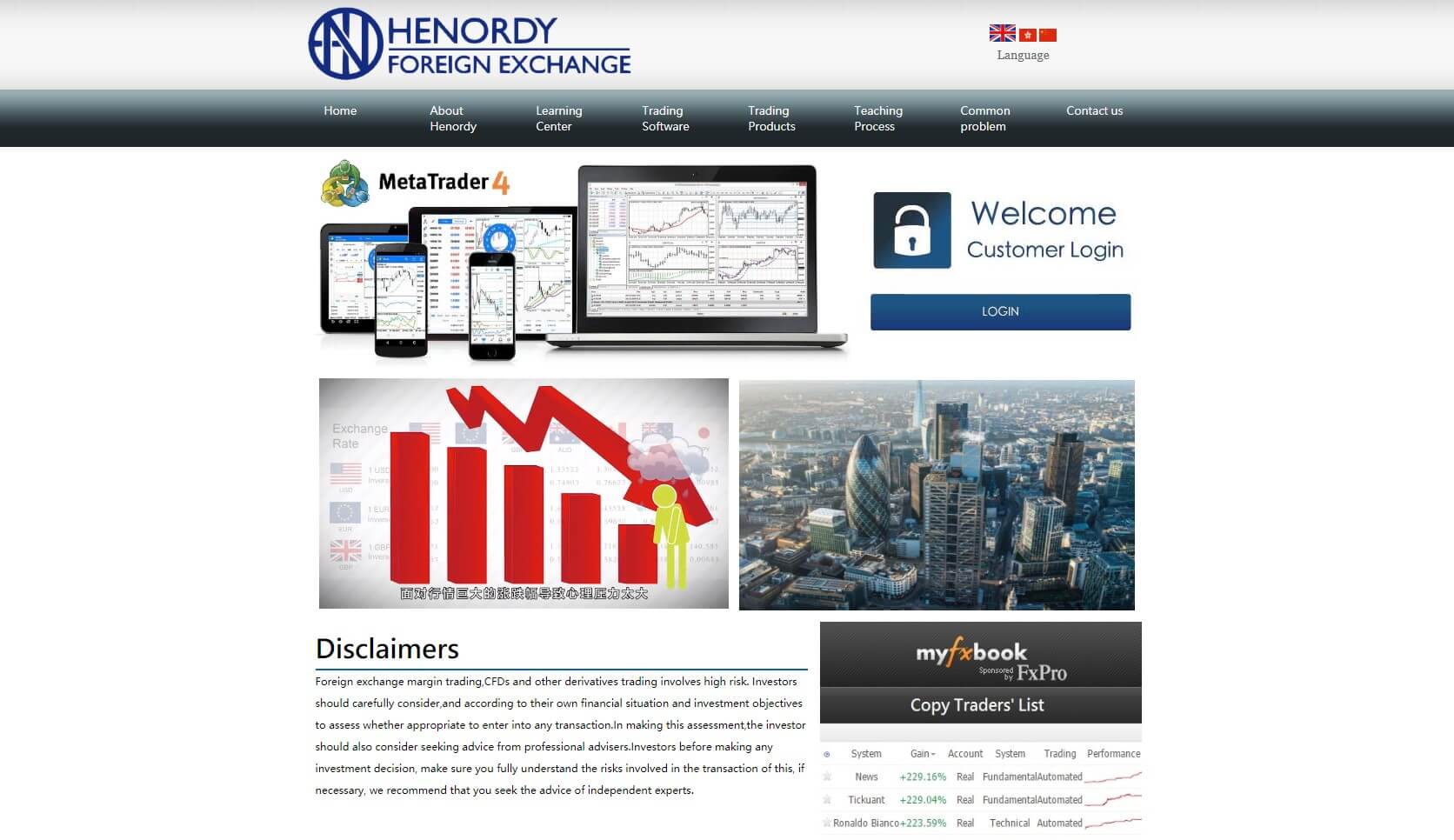The image is a detailed screenshot of a webpage. The top inch of the page is a nearly white, grayish strip. About two inches from the left-hand side, there's a dark blue circle with the letter "N" in its center, intersected vertically by a line that extends leftward from the circle. To the right of the circle, in all capital letters, is the word "HENORDY." A blue line appears below this, followed by the text "Foreign Exchange."

On the right side of the page, there's a prominent picture of the UK flag, about twice the size of other elements. Below it, there is a yellow flag featuring a central star, and another yellow flag with a star in the top left corner, labeled "Language" in black text.

Beneath this is a half-inch dark gray border. Following this, there are eight tabs for navigation, labeled "Home," "About Henry," "Learning Center," and so on, each guiding the user to different sections of the webpage.

In the main body of the page, on the left, there's an image of a person wearing a green shirt at the top, transitioning into a blue shirt in the middle, and a yellow shirt at the bottom. This person appears to be holding onto another person, viewed from a higher angle. Next to this image, the word "Metaphor" is written in black.

Further down, there are two laptops, with the one on the left being slightly smaller. In front of these laptops are two smartphones. To the right of this setup is another laptop computer. Adjacent to this is a blue square containing an unlocked white lock icon with the text "Welcome Customer Login" beside it. Below this, there is a blue button with the word "Login" in white.

Another section of the page depicts a declining money chart, with countries listed vertically on the left and decreasing red bars extending to the right. On the right side of the page, there's an aerial view of a cityscape. On the left side of this image, the word "Disclaimers" appears with approximately six lines of text below it. Additionally, on the right side, there are more gray boxes with various texts inside and below them.